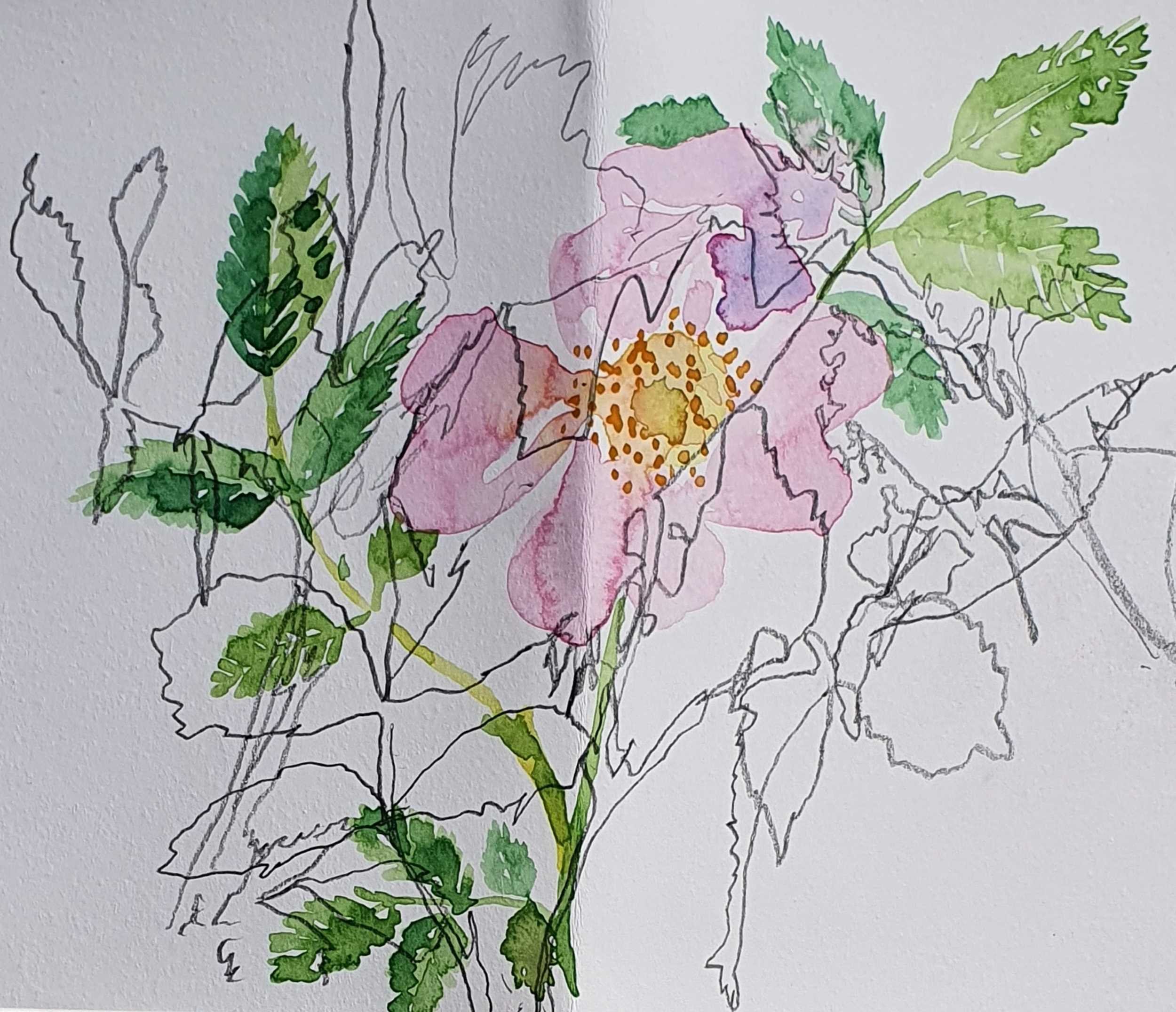The image depicts an intricate and partially colored illustration of a flower on a white paper background, which is slightly greyish with a noticeable crease running down the middle, suggesting it was folded at some point. Central to the composition is a detailed pink flower with a circular yellow center dotted with irregular brown and red spots. This primary flower features a mix of painted and unpainted petals, showcasing shades of pale pink, brown, and purple. The green stem of this flower extends upwards, surrounded by green leaves, some of which are painted in varying shades of green while others remain uncolored. Additionally, there is a secondary flower stem near the bottom left, with many sprouting leaves, also depicted in a mix of green and unpainted sections. The entire drawing appears to be outlined in black pencil, with some elements sketched more hastily yet artistically, adding a dynamic interplay between completed and incomplete artistic elements. In the background, the faint lines of another hastily scribbled flower can be seen, emphasizing the unfinished nature of the artwork. Overall, the illustration employs a color palette of green, brown, pink, purple, black, and white, harmoniously blending hand-drawn pencil outlines with vibrant colors and an unfinished aesthetic.